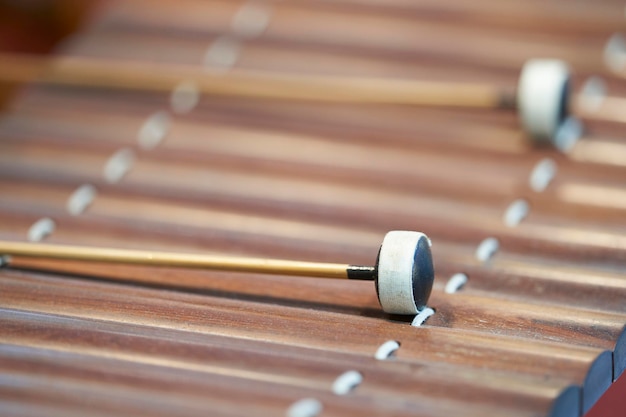The image is a detailed close-up of a wooden xylophone-like musical instrument, possibly a marimba or a set of woodpipes, used in various cultural contexts. The focus is on the upper section of the instrument where cylindrical wooden bars are clearly visible, though the background fades into a blur, obscuring the full structure. A dozen wooden bars can be seen, and they are interconnected by white lace or strings running down each side, holding the assembly together. Resting atop these bars are flat, round-headed mallets, reminiscent of Sweet Tarts, mounted on long wooden sticks. The mallet heads are black with white accents around the base, poised as if having just struck or about to strike the instrument. The scene lacks visible hands, directing all attention to the instrument and the striking tools.